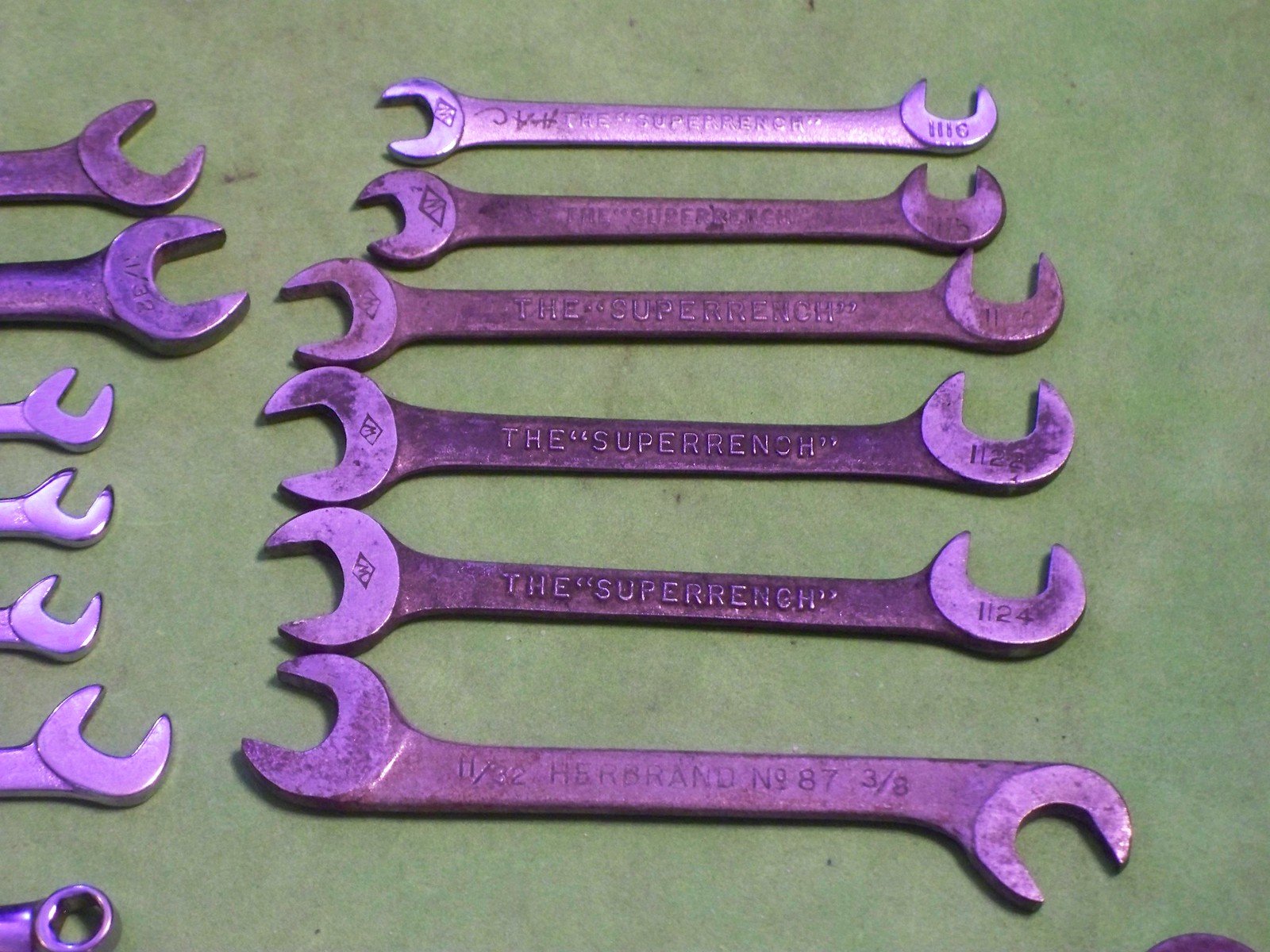The image showcases a collection of wrenches arranged on a greenish, light gray surface that appears to be a simple table or countertop. To the left side of the image, seven wrench heads are partially visible, their handles cut off by the edge of the frame. Dominating the center are six wrenches of varying sizes, all predominantly purple. Five of these central wrenches bear the brand name "THE SUPER WRENCH," with "SUPER WRENCH" etched into the metal in quotation marks. These wrenches also feature a four-digit code, such as 11-24, 11-22, down to 11-10, likely signifying their sizes. Despite their uniform purple appearance, they seem slightly aged and lackluster. Amongst them is one wrench that stands apart—a Herbrand wrench, marked with the size "11/32" and "3/8," hinting at its double-ended design. Some of the wrenches are adorned with initials, possibly engraved or written in marker, adding a touch of personalization to the otherwise industrial tools. The overall arrangement and the distinct color scheme make for a visually captivating and detailed display of these well-used, vintage wrenches.